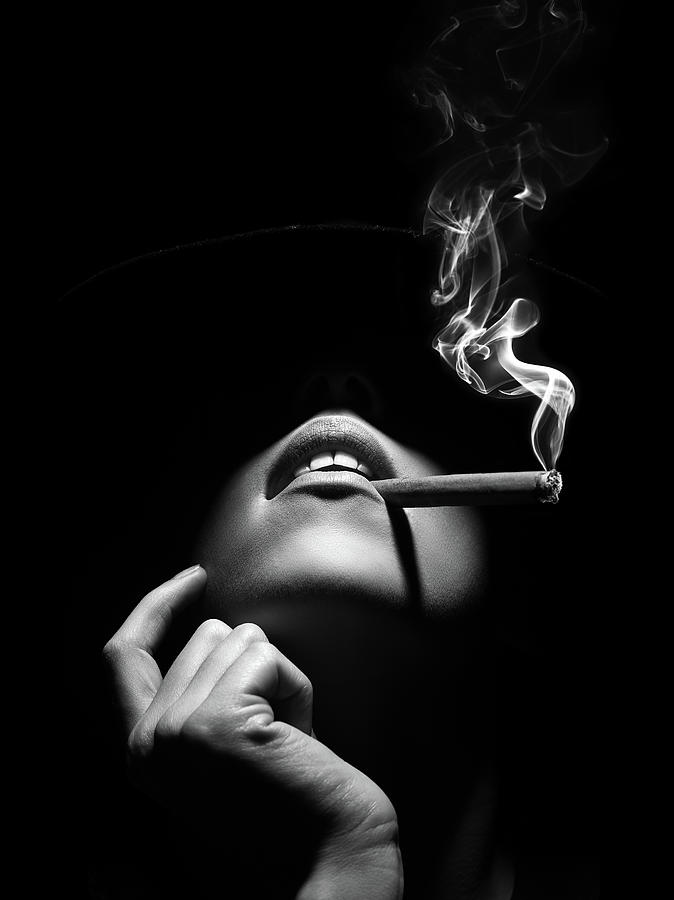The black-and-white photograph captures a striking close-up of a woman’s lower face, prominently featuring her chin, mouth, and the cigarette she’s smoking. Her smooth skin and expertly applied lipstick are visible, contrasting against a backdrop engulfed in deep shadows that obscure the rest of her face. The cigarette, appearing a rustic brown even in the monochrome palette, protrudes from the left side of her mouth with soft wisps of smoke elegantly curling up towards the top edge of the image. Her left hand is delicately positioned under her chin, with her index finger resting lightly on her cheek and the remaining fingers tucked beneath her jawbone, creating intricate, moody shadow play. The photograph’s high-contrast lighting and fast shutter speed have expertly frozen the motion of the smoke, adding to the artwork's professionalism and evocative allure. The entire composition, framed in a rectangular format, is a compelling blend of meticulous lighting and artistic expression, encapsulating a moment of serene sophistication in a beautifully crafted studio setting.